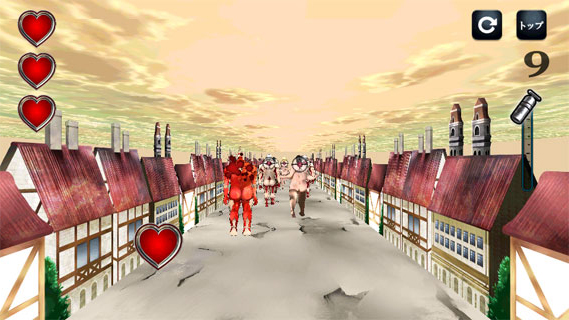In this vibrant, cartoon-style scene, numerous small structures resembling homes, barns, or businesses are neatly aligned on both the left and right sides of the image, creating a charming and bustling atmosphere. The center of the image features individuals walking towards the viewer, navigating the space between these structures. One particularly striking figure is entirely red, possibly a fantastical creature. On the left side of the image, three red hearts are vertically stacked, adding a whimsical and affectionate touch to the scene. The overall composition suggests a lively, game-like environment that one might encounter on TV or in an interactive game.